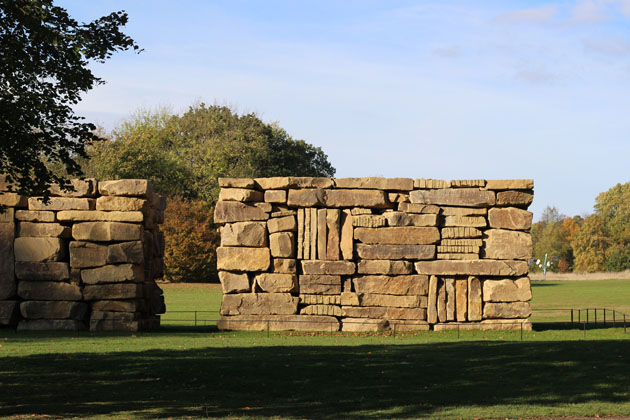The photograph showcases a significant stone structure reminiscent of Stonehenge, prominently situated within a sprawling park. The structure, composed of an arrangement of massive stones stacked both horizontally and vertically, stands as an imposing figure at an estimated height of 15 to 20 feet. Two primary stone formations are separated by a sizeable gap, creating a striking visual contrast against the expansive green field that surrounds them. The entire monument is enclosed by a black fence, clearly put in place to prevent close interaction and help preserve the integrity of this historical artifact. Positioned in the heart of the park, this stone structure serves as a focal point and a revered display, drawing visitors to observe and appreciate its grandeur from a respectful distance.